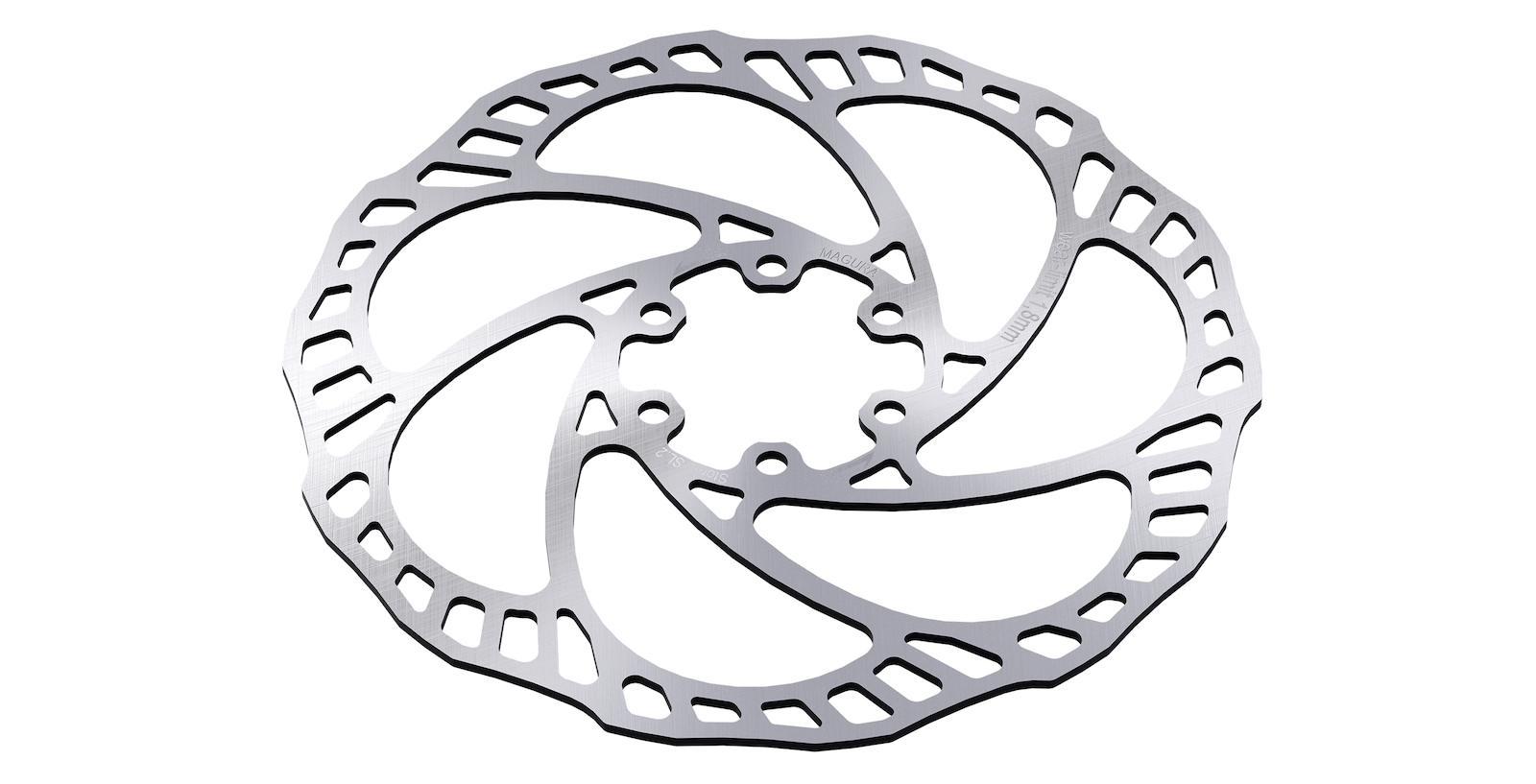This detailed digital rendering showcases a polished silver metal sprocket, characterized by its intricate and ornate design more suited for aesthetics than function. The circular machined part features a complex pattern that includes a central circle tied to an outer circle by spokes, creating a swirl-like appearance. The spokes spiral out almost tangentially, forming a dynamic radial pattern. The sprocket has multiple holes and cutouts, giving it a predominantly open structure where there is more void than material. The prominent perimeter is scalloped with hollowed sections that continue around its edge, adding texture and depth. Small mounting holes, six in total, are symmetrically drilled into the central circle, suggesting attachment points for assembly. Among the detailed cutouts are elongated teardrop shapes and triangles that intricately lace the inner region. Additionally, there is faint text on one part of the sprocket, including the notation "1.8mm." The background is pristine white, ensuring all elements of the metal's polished surface and intricate detailing are vividly highlighted.